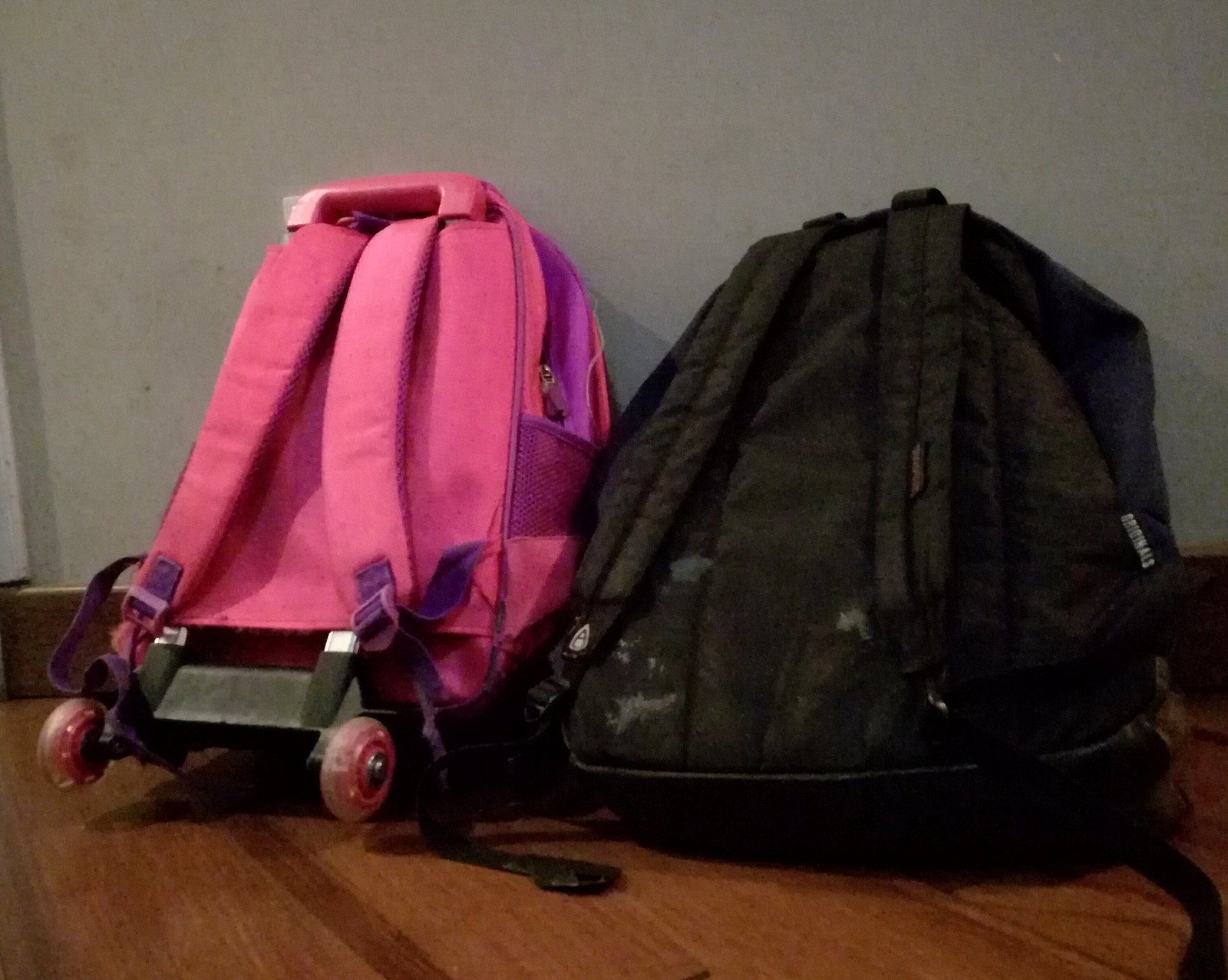This photograph captures two well-used backpacks resting on a wooden floor next to a white wall with a dark baseboard. The backpack on the right is black, featuring worn straps facing the camera and a sturdy, heavy-looking base that seems filled with items. The lower part of this black backpack shows noticeable wear, with some white staining indicating extensive use. Adjacent to it on the left is a pink backpack trimmed in purple, which doubles as a small suitcase with pink roller blade wheels attached to a metal frame. This pink bag is also positioned with its straps and a retractable pink plastic handle visible from the top. The wooden floor underneath highlights a blend of light and dark brown grains, adding a rustic feel to the background scene, while the white wall behind the bags provides a clean, simple backdrop to the well-traveled gear.